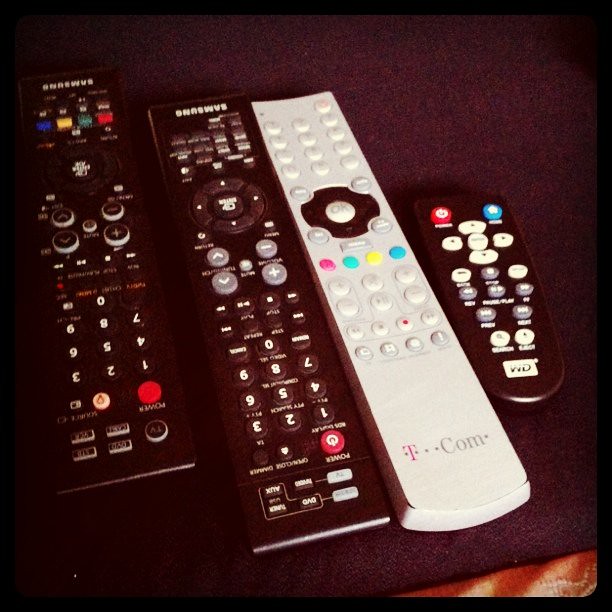A detailed photograph showcases four remote controls arranged vertically, with a slight angle, on a black surface that has a hint of brown at the front right edge. From left to right, the first remote is a long black Samsung remote featuring four colorful buttons at its base. Next to it, there is another Samsung remote, slightly smaller but also black, although the exact device it controls is unknown. The third in line is a long white remote labeled T-Mobile.com (or T-COM) at its base, adorned with various colorful buttons including pink, blue, and yellow. The smallest remote, located on the far right, is a compact black device with a WD (Western Digital) logo at the bottom, which likely belongs to a DVD player or a DVD-R recorder.